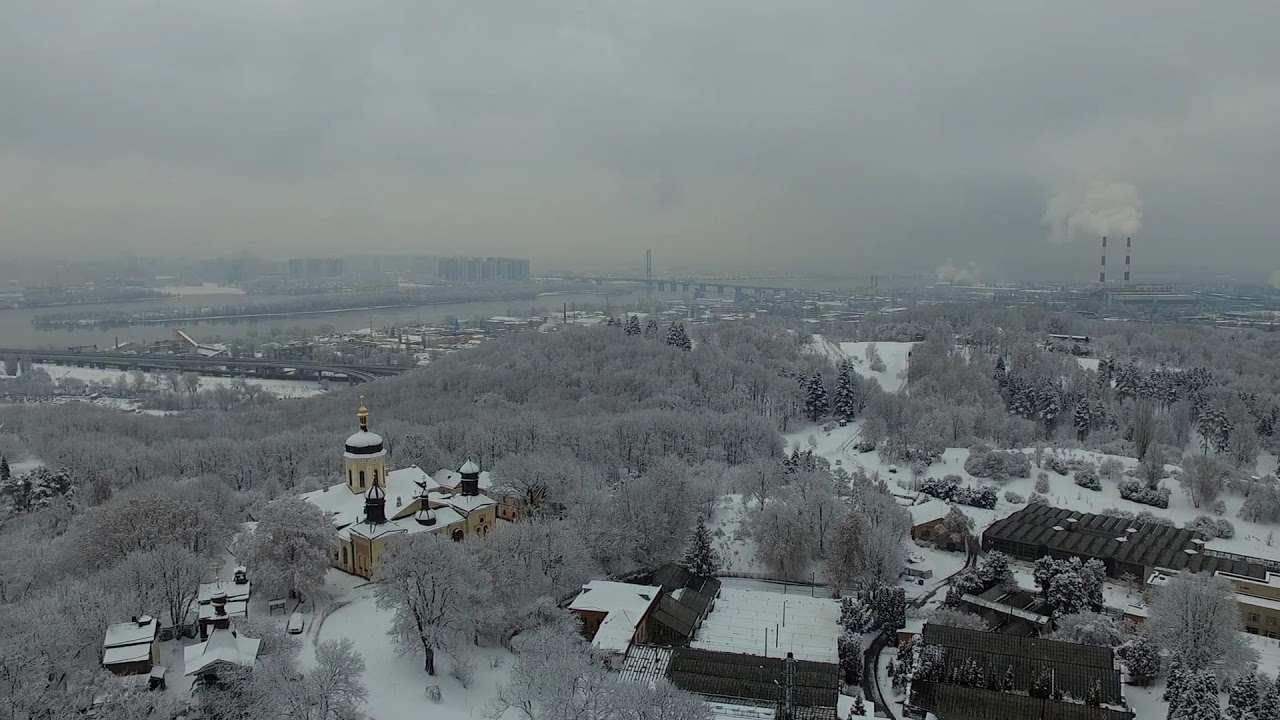The image portrays a winter landscape from an aerial viewpoint, either by drone or plane, capturing a town blanketed in snow. The scene is predominantly gray and overcast, lending a somber tone. In the foreground, frost-covered trees with a mix of white, gray, and hints of brown dominate, standing bare without leaves. The snowy ground enhances the wintry atmosphere.

Mid-ground features a cluster of buildings, including a prominent religious structure with domes, likely a church, and possibly a school or gymnasium, their rooftops laden with snow. Roads meander between these structures.

In the distance, a river bisects the town, crossed by a large bridge. On the riverbank, factories with red and white smokestacks release smoke into the polluted, cloudy sky, contributing to the grayish-brown hue above. Additional elements include apartment buildings faintly visible against the foggy backdrop, a harbor, and an island running through the river, adorned with trees and greenery. The entire setting is shrouded in a dense, grayish fog, creating a misty, wintry vista.